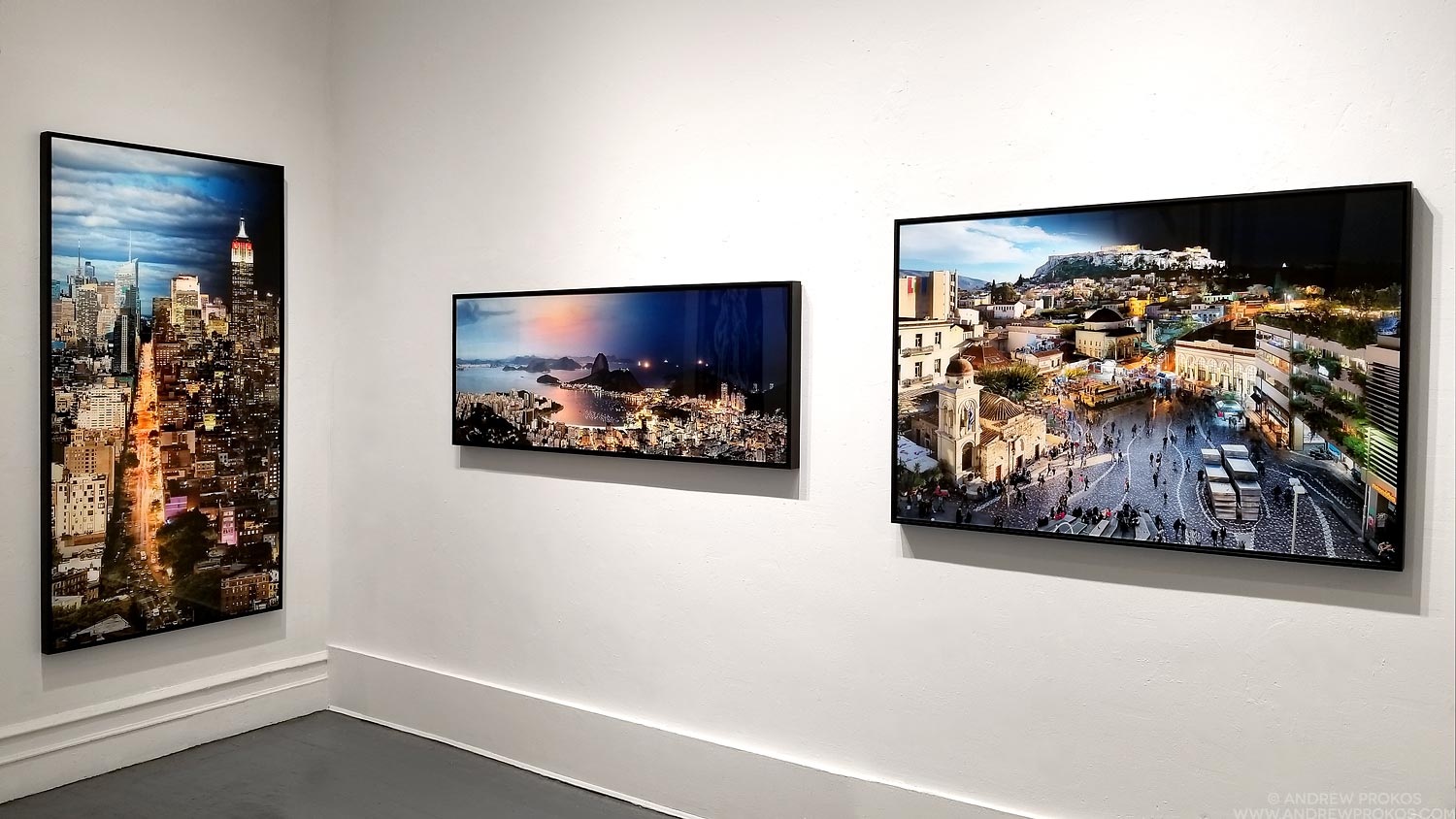This image captures a professional, museum-like gallery setting with a clean, sophisticated atmosphere. The backdrop consists of crisp white and grey walls that meet at a right angle, adorned with three large, framed aerial photographs, each vividly detailed and realistic. On the left wall hangs a substantial vertical print depicting a bustling cityscape, likely New York City, with towering skyscrapers, busy streets, and a vibrant blue sky. Adjacent to it on the right wall, two horizontal frames are displayed. The leftmost of these showcases a panoramic view of an island town, potentially along the Italian coast, featuring white buildings illuminated against a blend of blue sky and darkening night. The rightmost image portrays another dynamic city scene, highlighting a prominent tower amidst a myriad of urban details. Each photograph captures intricate elements such as people, historic architecture, natural landscapes, and coastal features, contributing to the overall professional and sophisticated ambience of the gallery.